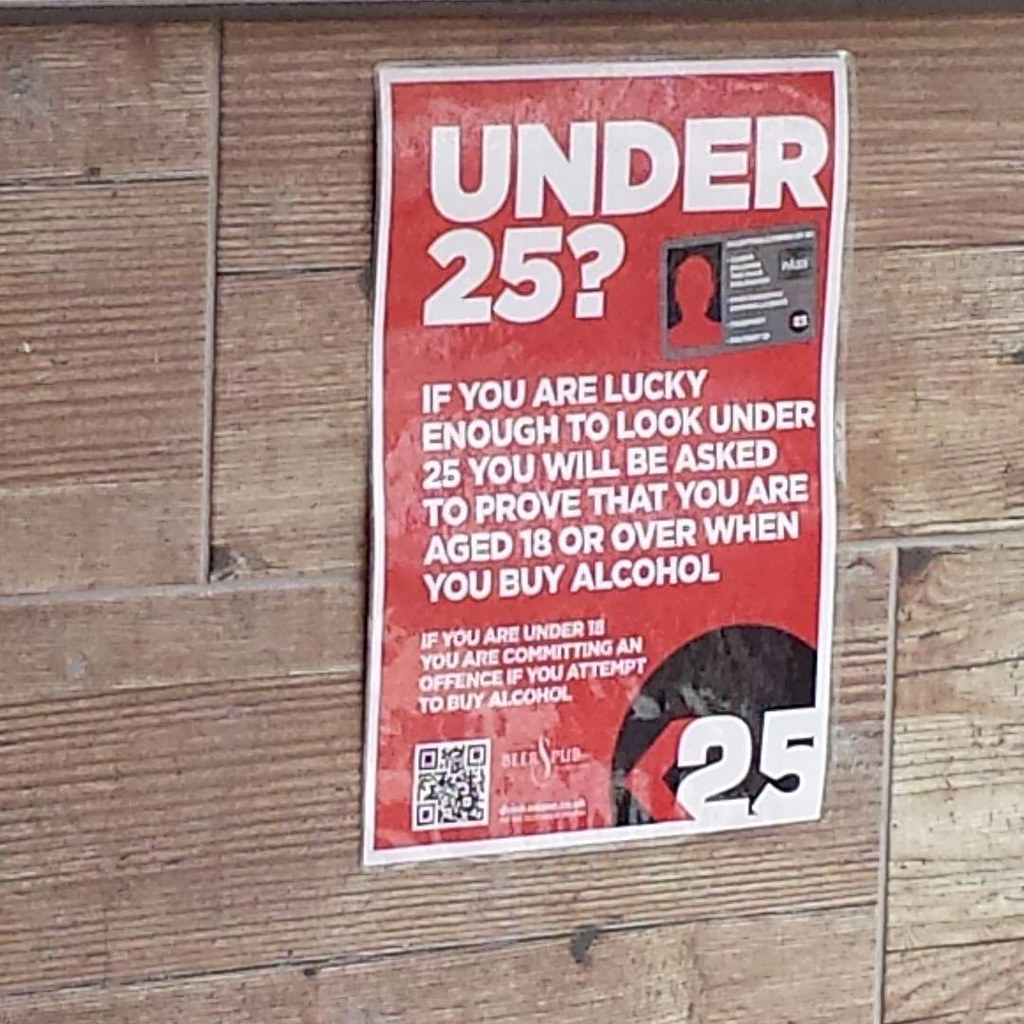The image depicts a laminated poster affixed to a wooden wall composed of several light brown, unevenly stacked wooden panels. The poster, positioned slightly off-center to the right, features a prominent white border framing its red background. At the top of the poster, large bold white text reads “Under 25?” followed by a gray ID card illustration with a human silhouette. Below this illustration, the poster contains several lines of white text: “If you are lucky enough to look under 25, you will be asked to prove that you are aged 18 or over when you buy alcohol” and further down in smaller letters, “If you are under 18, you are committing an offence if you attempt to buy alcohol.” On the bottom right corner of the poster, there is a black circular logo with the number 25 in large white font. Some other elements like a QR code and text reading “Bella's Pub” are partially visible but not fully legible.